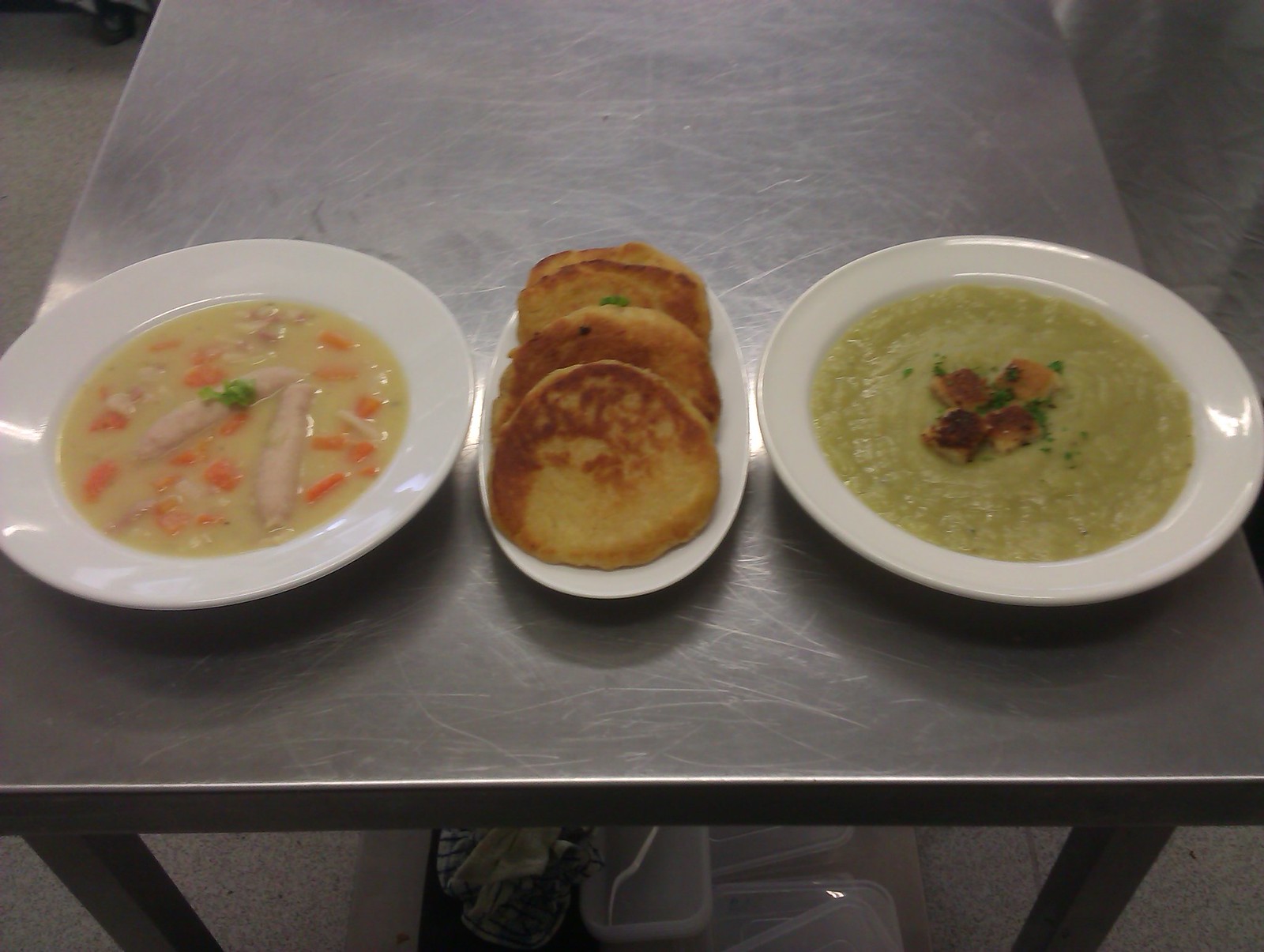The photograph captures a commercial kitchen setup with a scratched stainless steel table, featuring three distinct dishes. The table, supported by metal legs, has plastic containers barely visible underneath. Positioned vertically in the photo, the table holds two white ceramic bowls on either side and an oval platter in the center. The left bowl contains a creamy, chicken soup with orange carrots and pale pink sausages, garnished with green lettuce, with a wonton floating on top. The right bowl holds a thick, greenish pureed soup, possibly pea soup, with meat chunks sprinkled in the middle. The central oval platter displays three to four circular potato pancakes, partially stacked. The overhead angle of the shot provides a clear, detailed view of the meticulously arranged food on the metal surface.